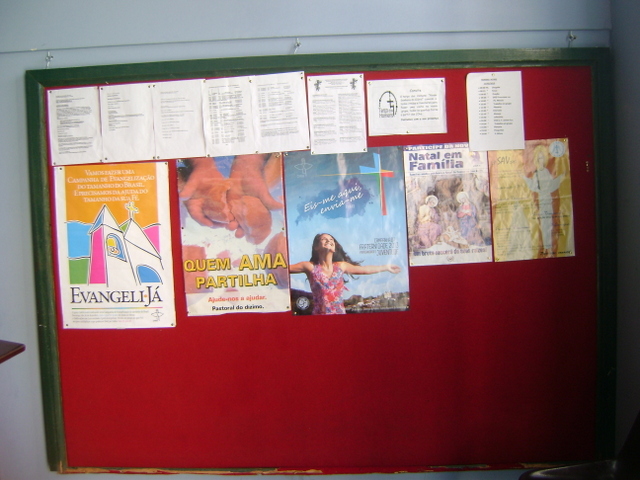This detailed color photograph captures a bulletin board hanging inside a church. The board itself is framed in dark green wood and covered with red felt. It is mounted on a white wooden wall, and its border is also trimmed in green wood. The board showcases a total of 13 pieces of paper or posters, arranged in a visually organized manner. The bottom section features five distinct posters, each displaying religious-themed images and messages. 

On the bottom left, there's an image of a white church with a crucifix on top and colorful windows in blue and pink. This poster includes the word "Evangeli-J-a" with a lot of unreadable text. Next to it, there's a poster depicting hands holding an indistinct object, possibly a tiny baby, highlighted by the yellow text "Q-U-E-M-A-M-A" and "P-A-R-T-I-L-H-A." The subsequent poster shows a blue background with a blue and red crucifix, featuring a young woman, likely between 20 to 30 years old, in a pink and red flowery dress, raising her hands in the air with buildings and trees in the background. Another poster displays the phrase "Natal-M-Familia," illustrating a nativity scene with baby Jesus, Mary, and either Joseph or one of the wise men. Finally, there's a gold-themed poster depicting a figure with arms raised, though the text remains indistinguishable. 

Above these are eight smaller, white papers with black text, likely scheduled events, announcements, or inspirational quotes, but their specific content is illegible. The overall scene suggests the board serves as an informative and inspirational centerpiece for churchgoers, emphasizing themes of faith and community.